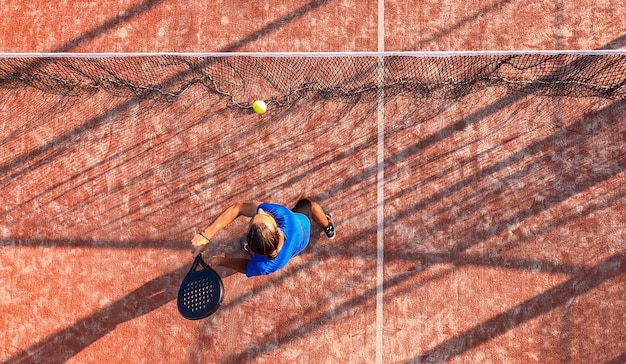The overhead photograph shows a man playing tennis on a dark red clay court, dotted with white spots and featuring a vertical white line in the middle. He is wearing a blue shirt and black shorts. The net, situated near the top of the image, appears loose and wavy, with a white top line and black netting below. The man is positioned with his right leg arched forward and is holding a black racket in his right hand, preparing to backhand a small yellow tennis ball that has just passed the net. The racket has small indentations in the center, giving it a unique texture.